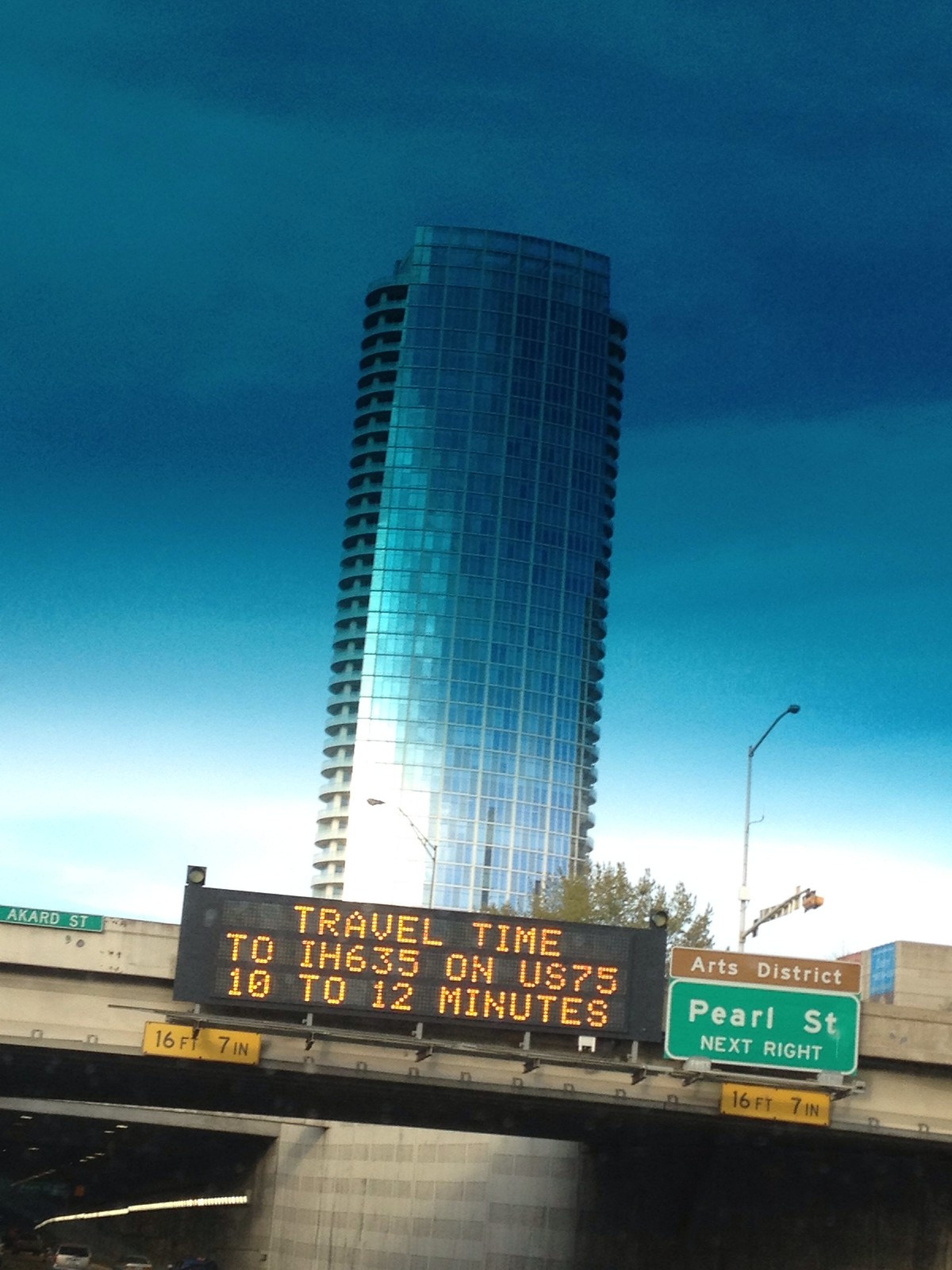The image showcases a towering skyscraper with a facade of mostly glass windows and metal framing, viewed from the perspective of a car approaching a highway overpass. The skyscraper, centrally located in the frame, features balconies on every floor and a blue, cloudy sky as a backdrop. The overpass spans a divided freeway, with the underside of concrete arches visible and a few distant cars cropped out of the image. Prominent street signage includes an electronic sign displaying "Travel time to IH 635 on US 75, 10 to 12 minutes" in orange-yellow text on a black background, and adjacent directional signs indicating the "Arts District" and "Pearl Street next right." The entire scene is slightly tinted blue, suggesting the photo was taken through the car’s windshield.